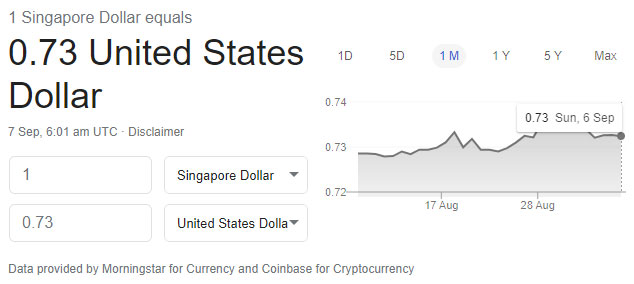This is a detailed screenshot of a Google currency conversion tool captured on September 7th at 6:01 AM. The tool indicates that one Singapore Dollar (SGD) is equivalent to 0.73 United States Dollars (USD), which is 73 cents. The interface displays two input boxes to allow users to select and convert between different currencies, with dropdown menus available for both choices.

On the right side of the screenshot, there is a small graph showing the fluctuation in exchange rates over various time periods including one day, five days, one month, one year, five years, and the maximum available range. The timeline on the graph spans from early August to August 28th, depicting minor fluctuations in the exchange rate without any drastic changes.

At the bottom of the screenshot, there is a disclaimer stating that the data for currency is provided by Morningstar, and for cryptocurrency, the data is sourced from Coinbase. This tool is useful for individuals who need to stay updated on currency exchange rates, whether for trading cryptocurrencies or other online transactions. This real-time data ensures users have the latest conversion rates at their fingertips.